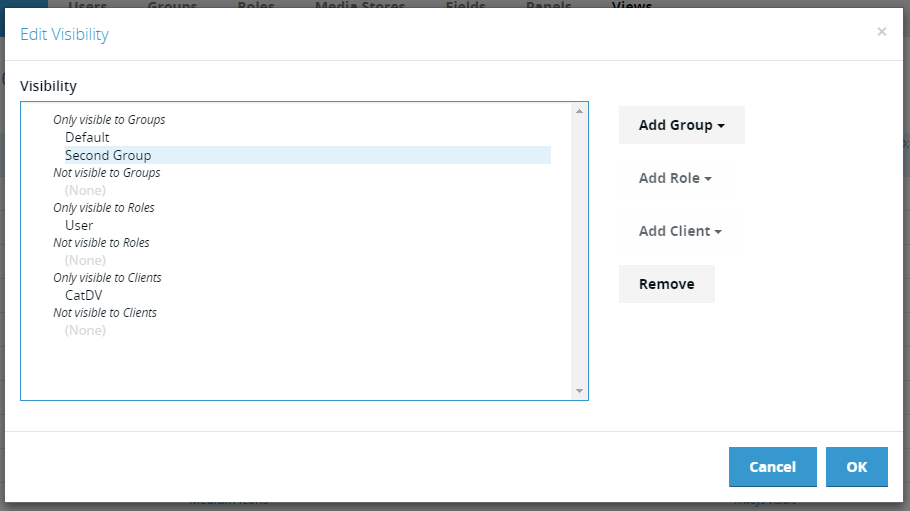The image depicts a gray rectangle measuring approximately six inches wide and three inches tall. In the top left corner of this gray rectangle, the phrase "Edit Visibility" is displayed in blue lettering. Below this header lies a smaller blue rectangle, nested within the larger gray rectangle. This blue box contains multiple visibility options, presented with specific criteria:

- "Only visible to groups"
- "Not visible to groups"
- "Only visible to roles"
- "Not visible to roles"
- "Only visible to clients"
- "Not visible to clients"
- "CatDV (Cat DV, a media asset management system), not visible to clients"

To the right of the blue rectangle, still within the gray boundary, are options for user actions. These actions include "Add a group," "Add a role," "Add a client," and "Remove." At the bottom of the gray rectangle are two buttons: a "Cancel" button and an "OK" button. It appears that this interface relates to editing visibility settings, possibly for users or content on a specific platform.